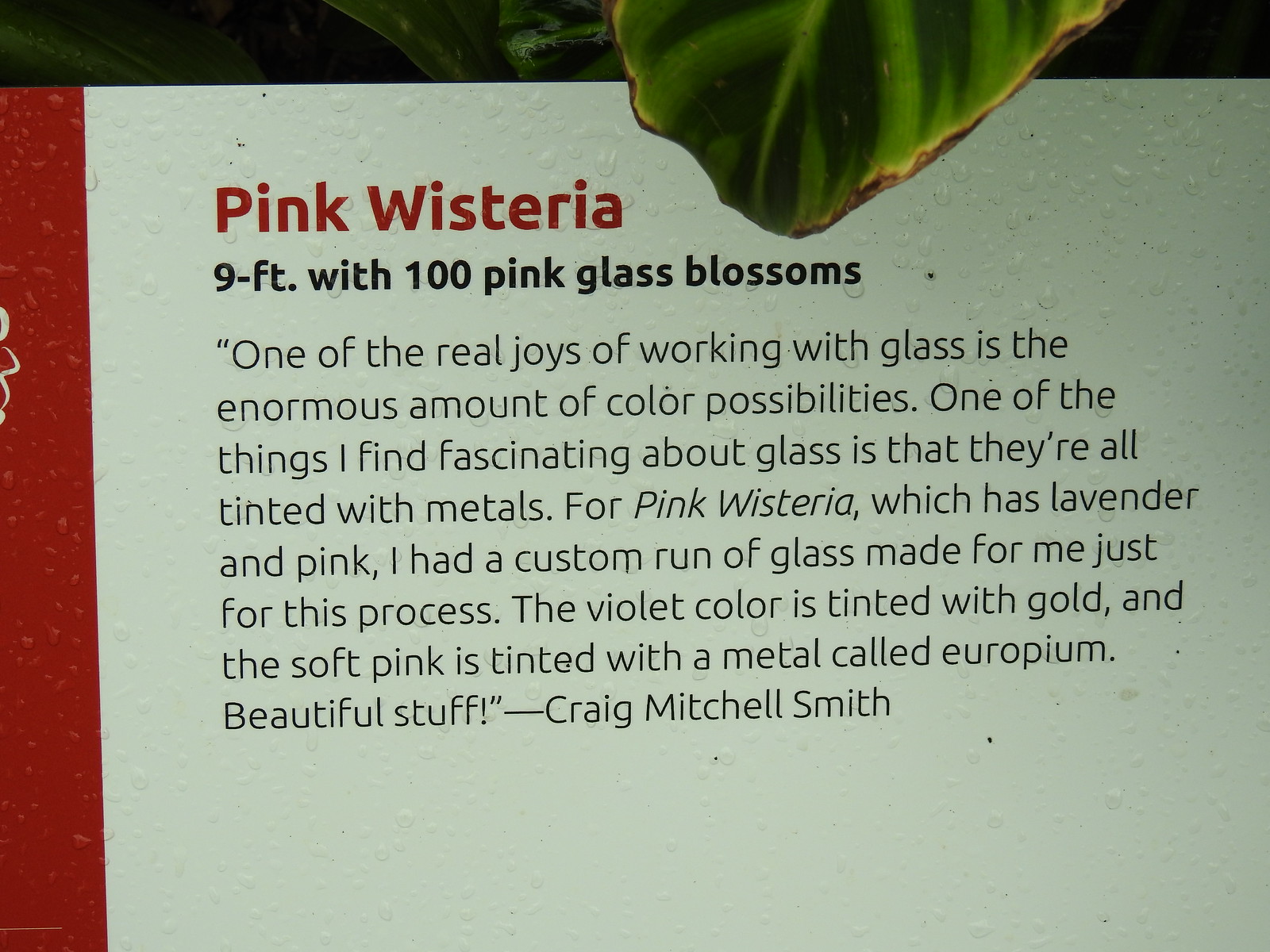The image shows a close-up of a sign titled "Pink Wisteria" with the text in red, P-I-N-K-W-I-S-T-E-R-I-A. This sign predominantly occupies the image and describes a nine-foot plant adorned with a hundred pink glass blossoms. The quote on the sign reads, “One of the real joys of working with glass is the enormous amount of color possibilities. One of the things I find fascinating about glass is that they are all tinted with metals. For Pink Wisteria, which has lavender and pink, I had a custom run of glass made for me just for this process. The violet color is tinted with gold, and the soft pink is tinted with a metal called europium. This is beautiful stuff.” The quote is attributed to Craig Mitchell Smith.

Visually, the sign is set against a white, possibly textured or slightly rain-speckled background, featuring a thin red strip along the left edge and a broader green strip with leafy textures running along the top. In the top center, a single green leaf is partially withered and shows signs of fertilizer burn. The surrounding environment suggests that the sign is located outdoors, likely in the middle of the day, and it displays a variety of colors including red, white, black, green, yellow, and brown.